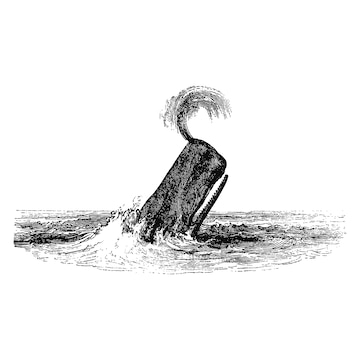This detailed etching, reminiscent of an 1800s illustration, captures the dramatic moment of a sperm whale breaching the surface of a calm ocean. The image, rendered in monochrome, shows only the whale's head emerging from the water. The whale is oriented to the right with an open mouth, exposing ridges suggestive of teeth, allowing the white background to be visible through the open jaws. Water arcs gracefully from near the tip of its nose, though oddly not from its blowhole. The splash around its body creates a dynamic interaction with the otherwise tranquil sea. Additional shadowing on the whale and patterning on the water enhance the realism, with small waves rippling in front of the whale and a notable cast shadow deepening the scene. The overall contrast of dark and light elements adds depth, making this very small piece a compelling and vivid portrayal of a breaching whale.